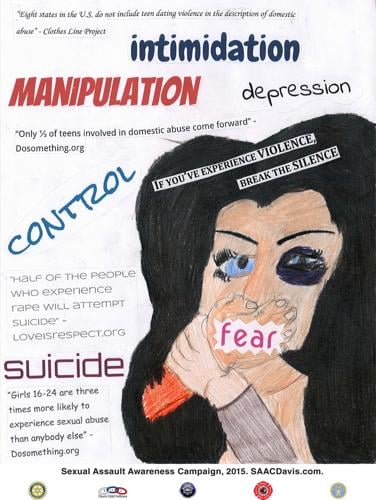This powerful magazine illustration features a young woman, drawn with a childlike crayon style, emphasizing the raw emotional impact of the image. The woman has black hair, and her eyes are mismatched: her left eye is blackened, presumably from a punch, while her right eye is blue. She covers her nose and mouth with her hand, and the word "fear" is boldly written over it.

The background of the image is filled with words such as "Intimidation," "Manipulation," "Depression," "Control," and "Suicide," reflecting the heavy themes of the artwork. Above her head, text reads, "If you've experienced violence, break the silence."

Several statistics are included in the image to emphasize the severity of the issue:
- "Girls 16 to 24 are three times more likely to experience sexual abuse than anybody else." (DoSomething.org)
- "Only half of teens involved in domestic abuse come forward." (DoSomething.org)
- "Half of the people who experience rape will attempt suicide." (Loveisrespect.org)

The image concludes with mentions of the Sexual Assault Awareness Campaign, 2015, and logos that are not clearly legible. This poignant public service announcement aims to raise awareness about teen dating violence and sexual abuse, urging victims to speak out.